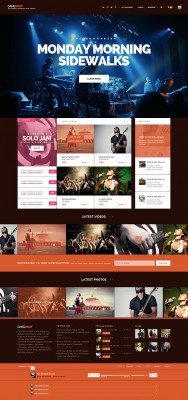In this image, a website is displayed on a cell phone. The top right corner of the screen features several small, indiscernible icons. Due to the image's small size, most of the text on the page is unreadable. The background of the website is predominantly black. Centrally positioned at the top is the phrase "Monday Morning Sidewalks" in white lettering. Below this text is a white button with black writing that remains too small to decipher.

The background image of the website shows a stage bathed in blue lighting, where people appear to be performing musical instruments. The picture is blurry and the specific instruments are unclear, though a drum set is vaguely noticeable on a stand.

Beneath this background image are four album covers arranged in the center, set against a white background with some accompanying text. Flanking these covers, one side features a pink background with the words "Solo Jam" in white, while the other side has an orange background with white writing.

Further down, there is a row of four or five images labeled with an orange tag containing white text. Below these are four or five more images, this time featuring a black box with additional images. At the very bottom of the page, there is another orange box with white writing.